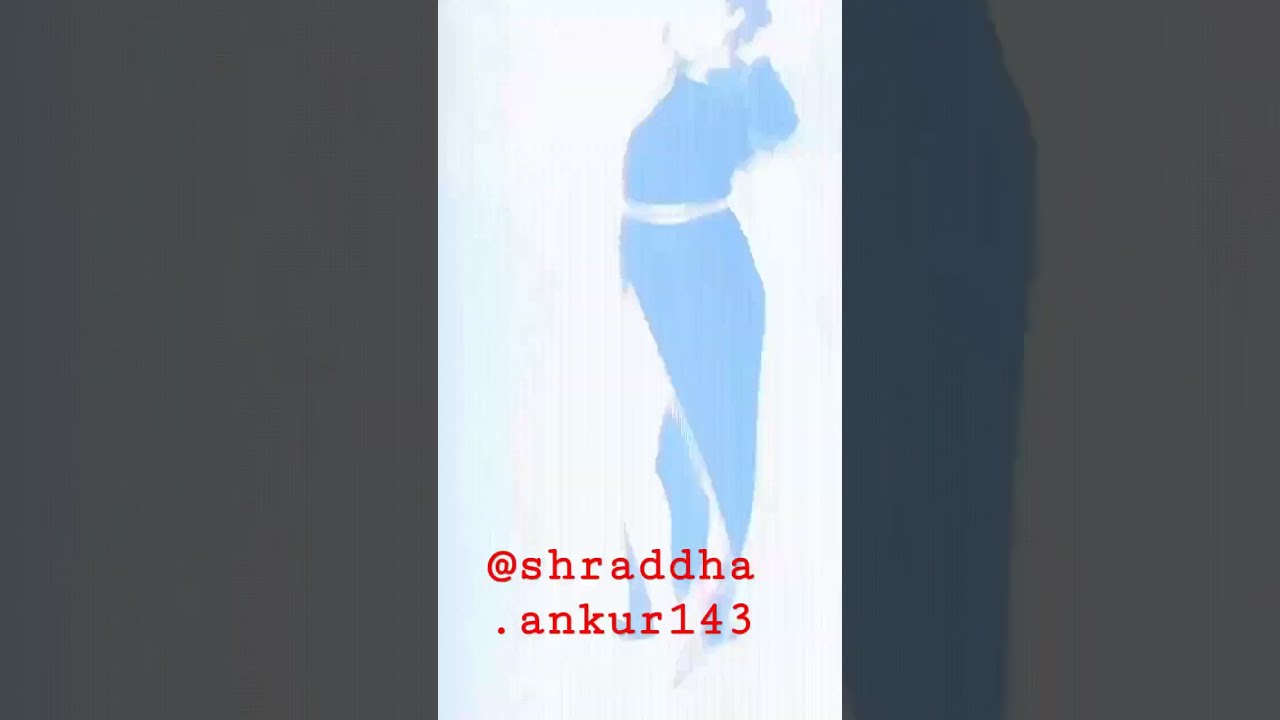The blurred image centers on a woman with short dark hair, wearing a long dress with a high slit on her right thigh. The dress appears to be dark in color, contrasted by a lighter-colored belt. Although the image is highly overexposed and out of focus, making details difficult to discern, the background is predominantly white with light blue accents on either side. The picture is divided into three vertical sections: the left and right sections are much darker, while the middle section, where the woman is depicted, is brighter. The text "at shrada.ankar143" is printed in red at the bottom of the image. The entire composition is enveloped in various shades of gray, purple, light blue, and white, adding to its complexity and obscurity.